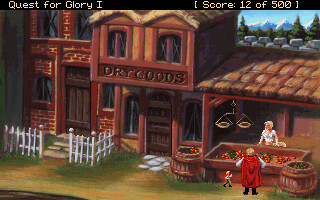This image appears to be a still from a video game titled "Quest for Glory I," as indicated by the text in the top left-hand corner. The score of 12 out of 500 is also displayed on the top right-hand side. The scene is set in an old-school town comprising two two-story buildings made of brown and red bricks, with wooden doors and windows on both levels.

The first building on the right has a small white gate and a sign on the upper level that reads "dry goods." Adjacent to this building is a small market stand with a shelter, where a woman stands behind the counter displaying fruits and vegetables, along with a weighing scale. Across from her, a man in a red cape, accompanied by a little boy, appears to be examining the produce. A large barrel stands nearby them.

In the background, there are snow-capped mountains and a clear blue sky, adding a sense of tranquility to the scene. The detailed setting, vibrant characters, and scenic elements contribute to an immersive and picturesque depiction of this game environment.